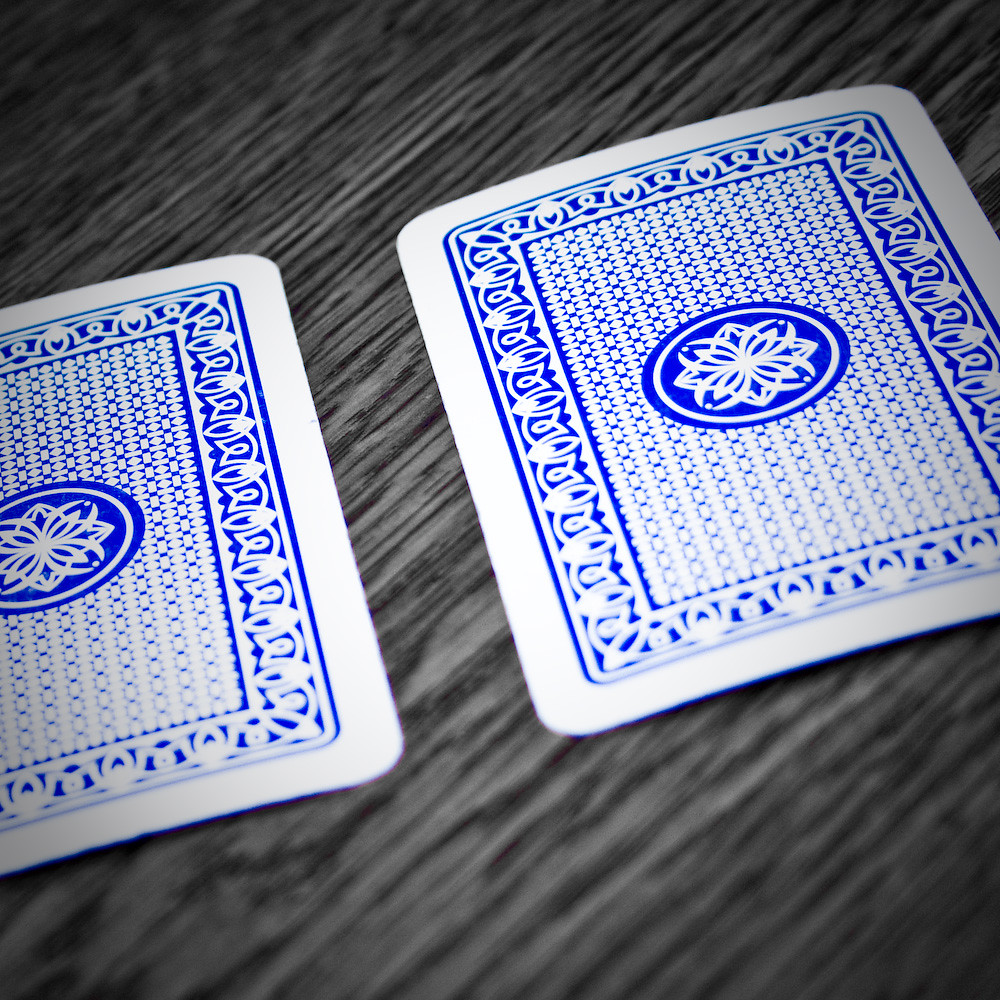In this meticulously detailed close-up image, two playing cards are laid out on a weathered gray wooden table, marked by numerous cracks and crevices that suggest years of wear. The cards, by contrast, are nearly pristine, indicating minimal handling. The card on the left occupies approximately 60-75% of the frame, while the card on the right is roughly 75% visible, with its bottom left corner out of sight.

Both cards feature a striking blue and white design. The outer border consists of repeating elongated shapes reminiscent of curly cues or abstract eye-like forms. Within this border, a more intricate pattern dominated by spiky figure eights arranged in a grid fills the central area, giving the impression of fine fabric stitching. At the very center of each card lies a series of concentric circles: a blue outer ring, a white circle, and a solid blue inner circle adorned with a white spirograph motif. This central design evokes an intricate diamond or butterfly shape, adding to the visual complexity. The cards are face down, leaving their identities a mystery.